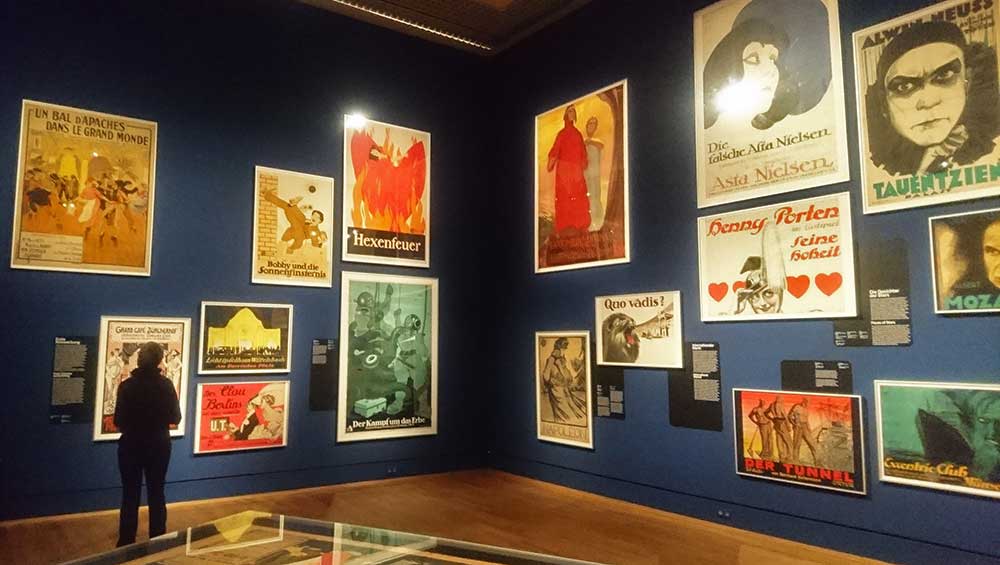In this image, a person dressed in black stands towards the bottom left side of a vast art gallery or museum, their silhouette framed against the dark navy walls. The wooden floor beneath them is polished and contrasts with the room's overall dim ambiance. On both the left and right walls, an array of framed posters is visible, though many are difficult to read due to their distance. Some discernible titles include "Aston Nielsen," "Eccentric Club," "DER Tunnel," and "Hexenfuehrer," with informational black cards adjacent to them, though their text remains unreadable. A display case corner is also visible in the bottom left, made of glass and containing unidentified objects. The ceiling peeks into the top middle of the frame, revealing a dark gray hue, adding to the room's sombre yet sophisticated atmosphere.